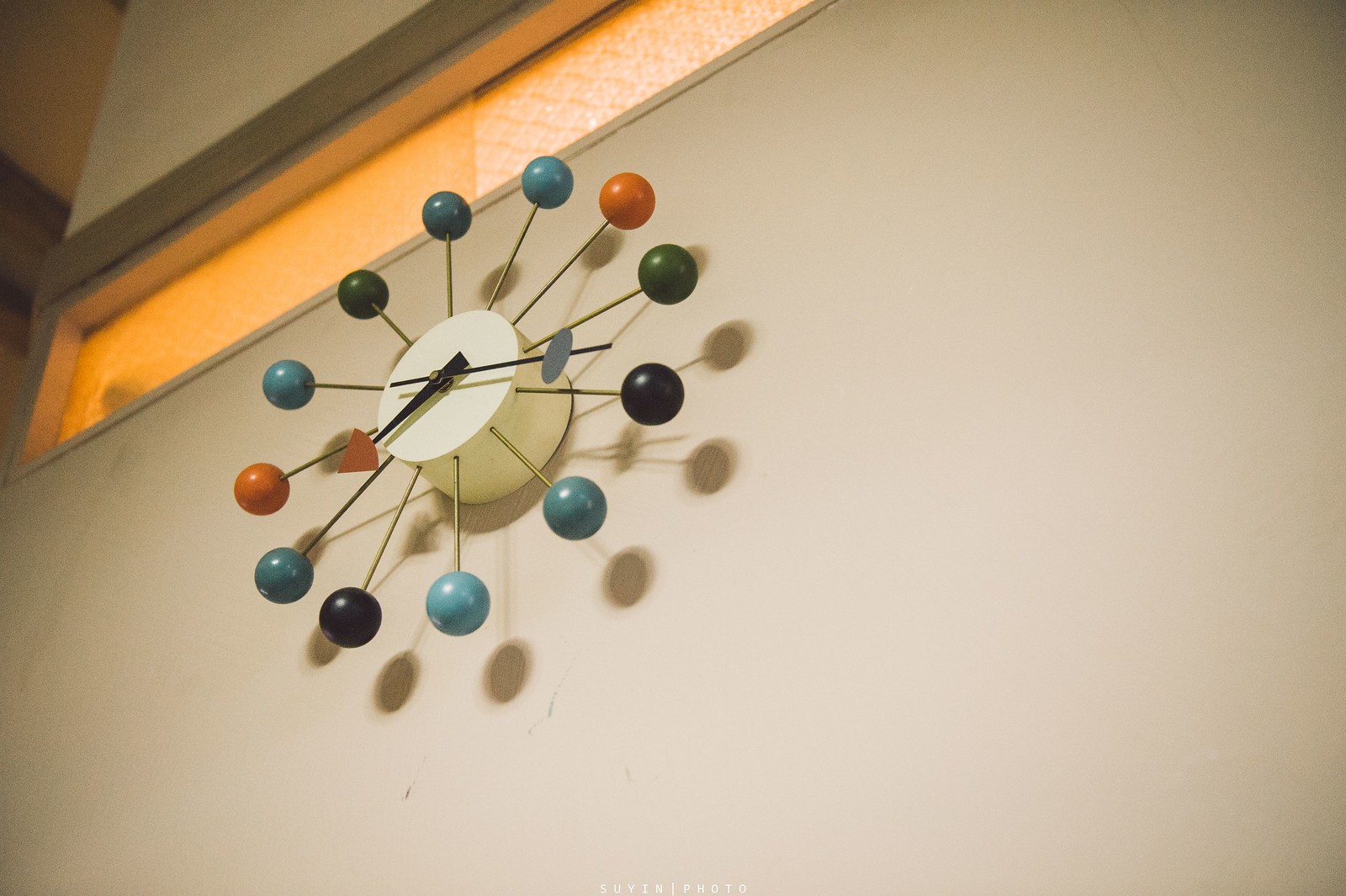An upward-angled view of a modern, stylish clock features prominently in the image. The clock is distinctive with its unique design, showcasing a series of colorful balls mounted on thin metal rods arranged in a radial pattern around the clock's center. These balls, representing the hours, are color-coded and positioned at the traditional intervals of 5, 10, 15, 20, and so on up to 60 minutes. 

The central element of the clock face is a small, thick white circle from which long black hands extend. The hour hand is characterized by an orange triangle at its tip, while the minute hand is marked with a gray oval. This contemporary clock is mounted on an ivory-colored wall, above which there is a large rectangular window fitted with frosted orange glass, adding a touch of warmth and color to the setting.